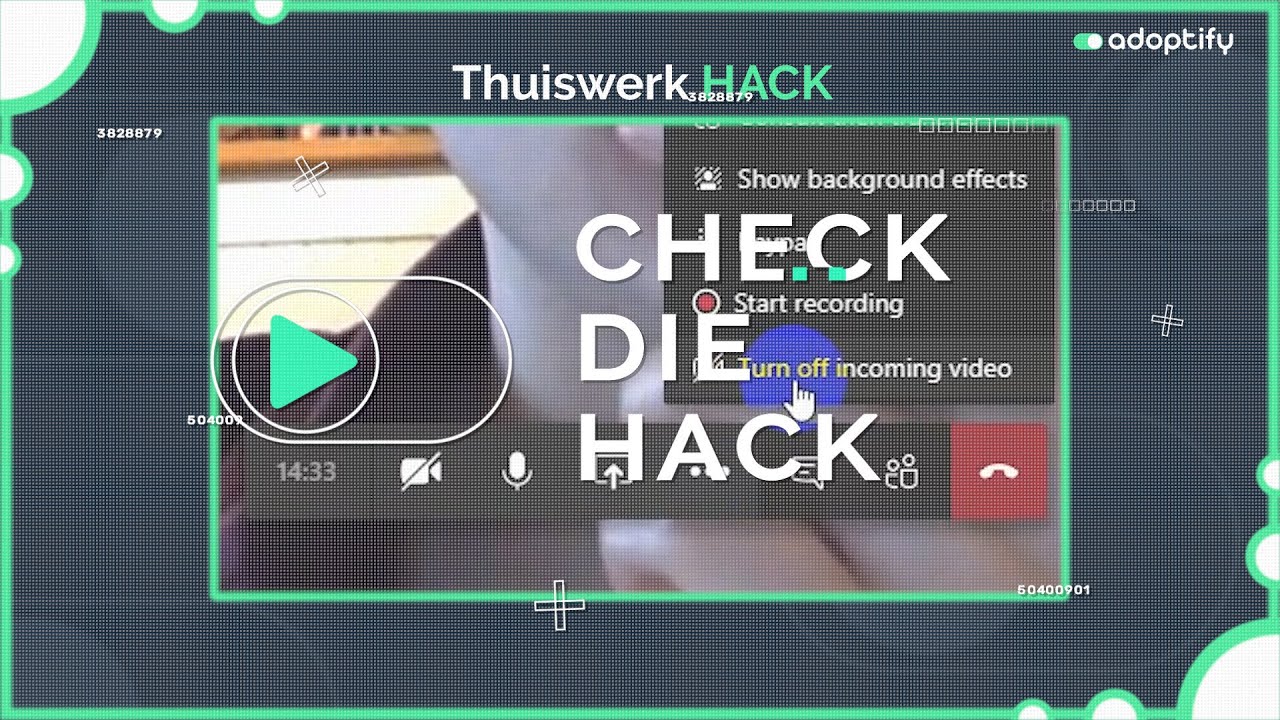This image is a detailed screenshot from a website, featuring a predominantly dark blue background with a light green border. Within this border, a smaller rectangle displays an unclear image overlaid with a large green play button. At the top right corner of the image, the logo "Adoptify" is visible. Centrally positioned at the top, the text "THIUSWERK" appears in white, followed by the word "HACK" in uppercase, colored light green.

The central image, seemingly a thumbnail, displays the phrase "Check DIE Hacks," likely hinting at German origin. This thumbnail suggests it is the start of a video, illustrated by the prominent play button. Behind this image, additional interactive elements are visible: the options "Show Background Effects," "Start Recording," and "Turn Off Incoming Video," reminiscent of a video conferencing interface. Further, partially obscured symbols include a countdown timer showing "14:33," a camera icon with a slash through it, a microphone symbol, and a telephone symbol within a red square, indicating typical controls found in platforms like Zoom or Microsoft Teams. The entire setup seems to be a product demonstration, possibly offering video call features.